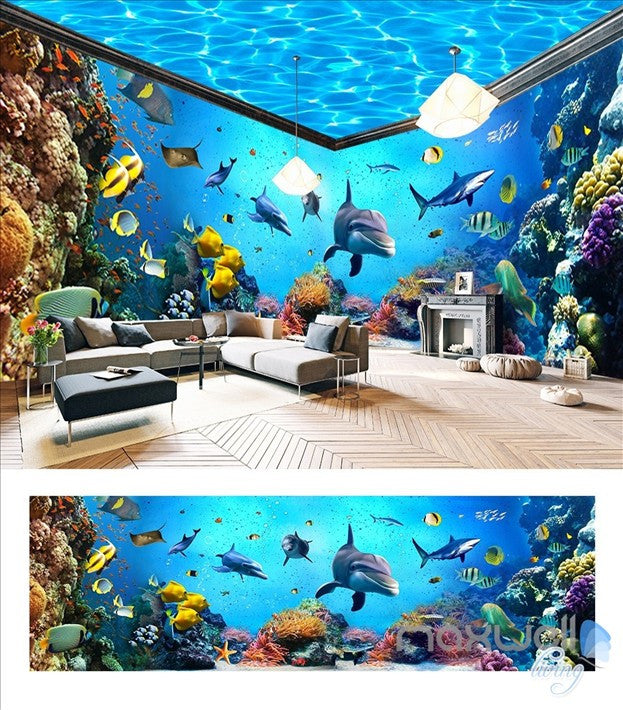This image showcases an intricately decorated living room with an oceanic theme. The room appears to be an artistic blend of real and fantastical elements, highlighted by vibrant, cartoonish wallpaper that makes it look like you're submerged underwater. The wallpaper features an abundant array of sea creatures, including dolphins, sharks, and tropical fish, majestically weaving through colorful coral.

The living space itself is furnished with cozy elements, including a couple of plush couches adorned with pillows, a wooden table, and lush green plants. To the right, there's a fireplace adding a touch of warmth to the underwater illusion. The floor is wooden, topped with a white rug that contrasts against the vibrant hues of the oceanic backdrop. Hanging lights are suspended from a ceiling that has been masterfully painted to resemble the shimmering surface of a pool, creating an immersive effect of being beneath the waves.

The overall setting is a mind-blowing fusion of reality and fantasy, with the room's decor seamlessly merging with the vibrant and dynamic ocean scene. The colors in the room span a stunning spectrum of blues, yellows, oranges, browns, tans, grays, and whites. Additionally, a mysterious cave door is visible to the right, further enhancing the whimsical, underwater ambiance. This imaginative and high-quality decoration truly transforms an indoor space into an enchanting underwater paradise.